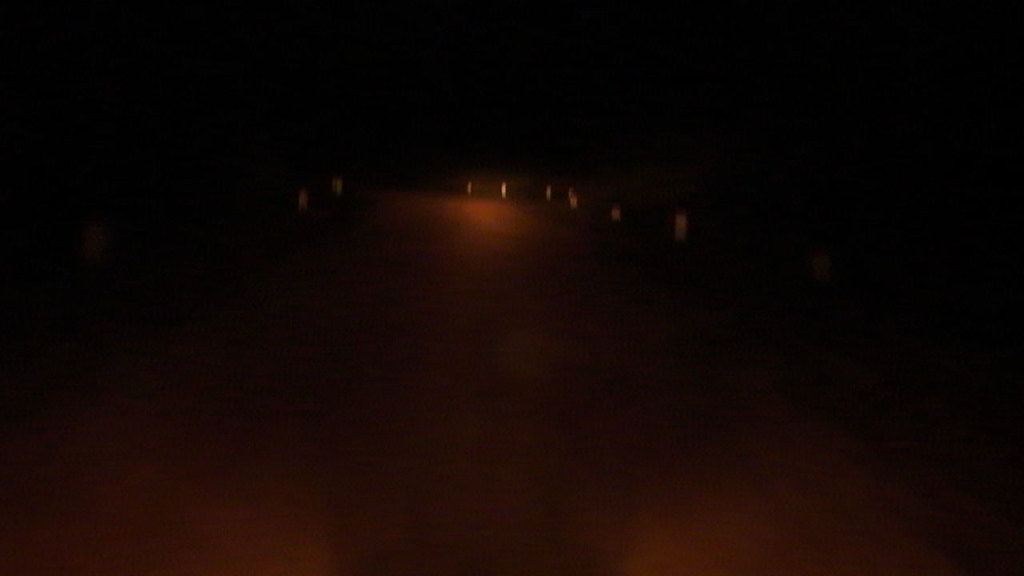This image depicts a scene shrouded in darkness, with the upper portion fading into pure black and gradually transitioning to very dark reds and browns towards the bottom. Centrally, there is a diffuse, slightly illuminated area with a notable small, red brighter spot. Across the middle of the image, thin vertical lines stretch from left to right, resembling either stakes or signs that hint at a roadside setting. These faint markers, which appear white or yellow, suggest the presence of a road, possibly indicating its edges or a curve. The light seemingly emanates from a distant source, causing a subtle gradient from the dark foreground to the lighter background. This light casts just enough illumination to create blurry blotches of brown, hinting at possible hedgerows or vegetation, although the low lighting conceals most details. The overall impression is that of a nighttime scene, potentially viewed from within a vehicle, with the light source being headlights reflecting on the road surface, giving the otherwise pitch-black surroundings a faint, eerie glow.